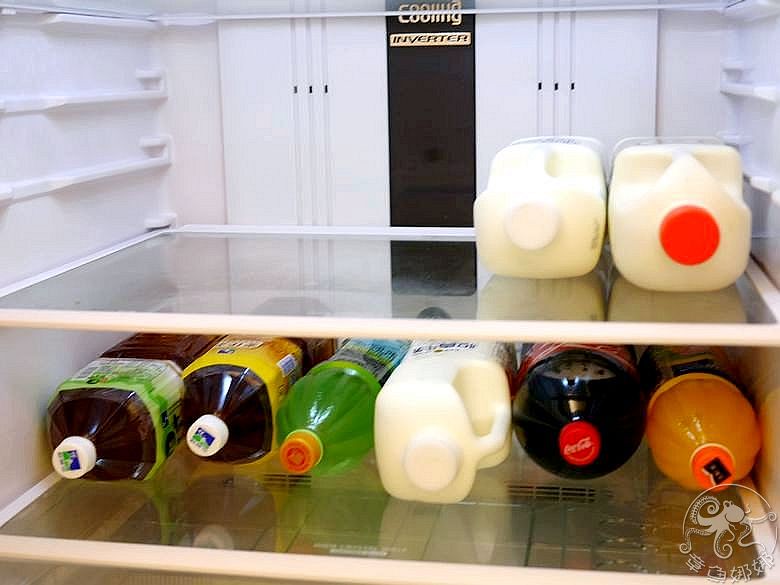This photograph captures the contents of an open refrigerator, focusing on its top two shelves. The refrigerator is white, and both shelves feature various beverages. On the top shelf, there are two jugs of milk lying on their sides with the caps facing the camera. The jug with a white cap is slightly smaller, while the larger jug has a bright red cap. The second shelf is crowded with an assortment of drinks. On the left, there's a slightly larger juice container with a green label, and next to it, a smaller juice container with a yellow label. There is also a green bottle containing a clear liquid, possibly sparkling water or soda, with a red cap. In the middle of this shelf is another jug of milk with a white cap. To the right of the milk, there's a two-liter bottle of Coca-Cola with its characteristic red cap and logo. Adjacent to the Coca-Cola is a bottle of orange juice or another type of citrus drink with an orange cap and a logo. At the bottom right hand corner of the refrigerator door, there is an octopus symbol along with text in a different language, possibly indicating a trademark or watermark. Outside the refrigerator is a black strip labeled "cooling inverter."